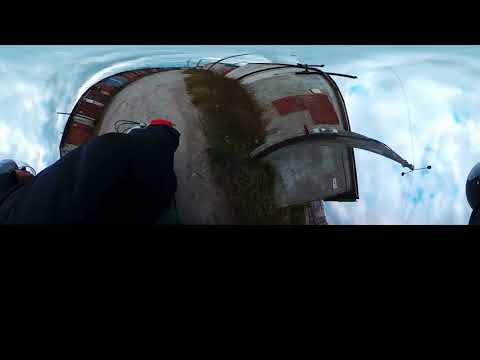The image captures a slightly blurry and distorted outdoor scene, seemingly taken with a fisheye lens, which warps the visuals dramatically. Dominating the image is a small, gray, rounded structure featuring a metallic, cement-like body, with a smaller, similar shaped attachment. Wrapped around this structure are green, grass-like elements, suggesting some foliage present. The sky above is a vivid blue interspersed with white clouds, casting daylight across the scene and enhancing the bright, overall setting. In the background, one can glimpse what appears to be an alleyway or an unpaved dirt road, indicating a rural or less urbanized part of town. To the left, a figure dressed in a black jacket with red gloves is either walking or riding a motorcycle on this path. Additionally, on the far left side of the image, there is a black protruding object, likely a tower or a utility pole, and on the right, a shiny black spherical element, perhaps a component of the structure or a reflective object, is visible. The overall scene merges shades of gray, green, black, and blue seamlessly, conveying a dynamic and somewhat surreal environment.